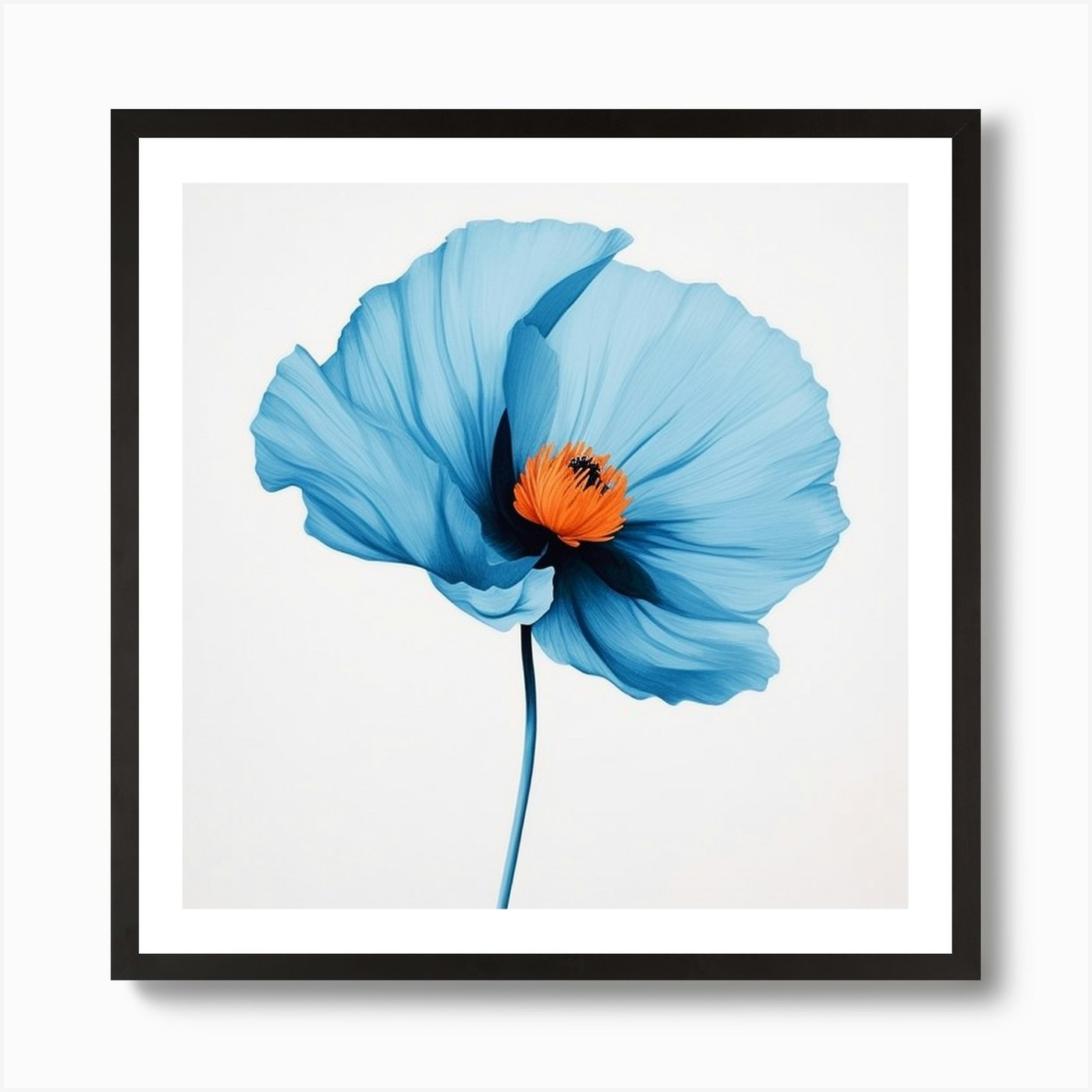The image features a large framed painting of a striking blue poppy flower with a blue stem, set against a light gray to almost white background. The flower’s silky, thin petals radiate outward from an orange and black-shaded center, giving it a dynamic, almost gown-like appearance. The realistic yet clearly painted flower dominates the canvas, showcasing the vibrant blue hues that contrast beautifully with the orange stamen at its core. The painting is bordered by a white mat, all enclosed within a black frame. This elegant framed artwork is mounted on a white wall, likely resembling a gallery setting, with the frame casting a subtle shadow that enhances its presence.